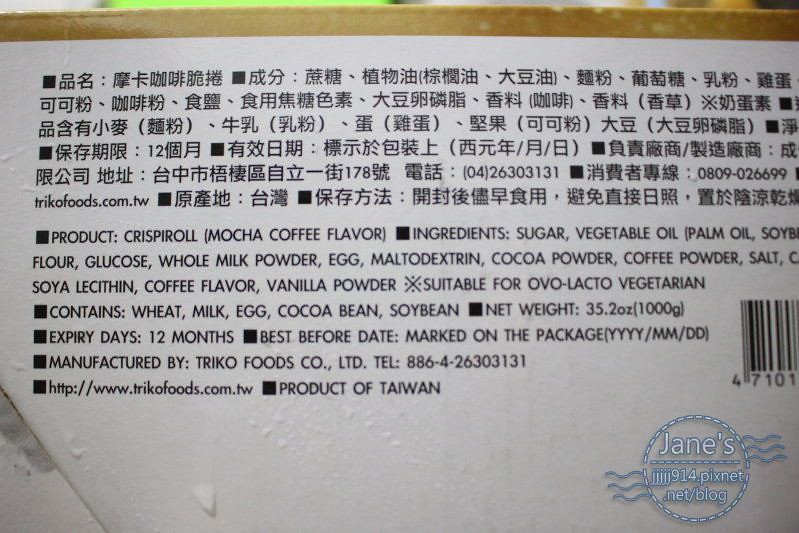The color photograph depicts the back label of a packaged food product on a white background. The top third of the label features six rows of what appears to be Chinese or Taiwanese text. Below this, the English section of the label begins with a black square followed by the product's name: "Product: Crispy Roll (Mocha Coffee Flavor)." Another black square introduces the ingredients list, which includes sugar, vegetable oil (palm oil, soy), flour, glucose, whole milk powder, egg, maltodextrin, cocoa powder, coffee powder, salt, soya lecithin, coffee flavor, and vanilla powder. Additionally, there's a symbol indicating the product is suitable for ovo-lacto vegetarians. The label also states that the product contains wheat, milk, egg, cocoa bean, and soybean.

Further down, there are black squares indicating various details, including the net weight of 35.2 ounces (1,000 grams), and another marking for 12 ounces. The best before date format is indicated as YYYY/MM/DD. The manufacturer is listed as Trico Foods Co. Limited, with a contact number of 886-4-263-03131, and a website at "http://www.tricofoods.com.tw." The label also states the product is of Taiwanese origin. To the right of these details, there's a UPC label.